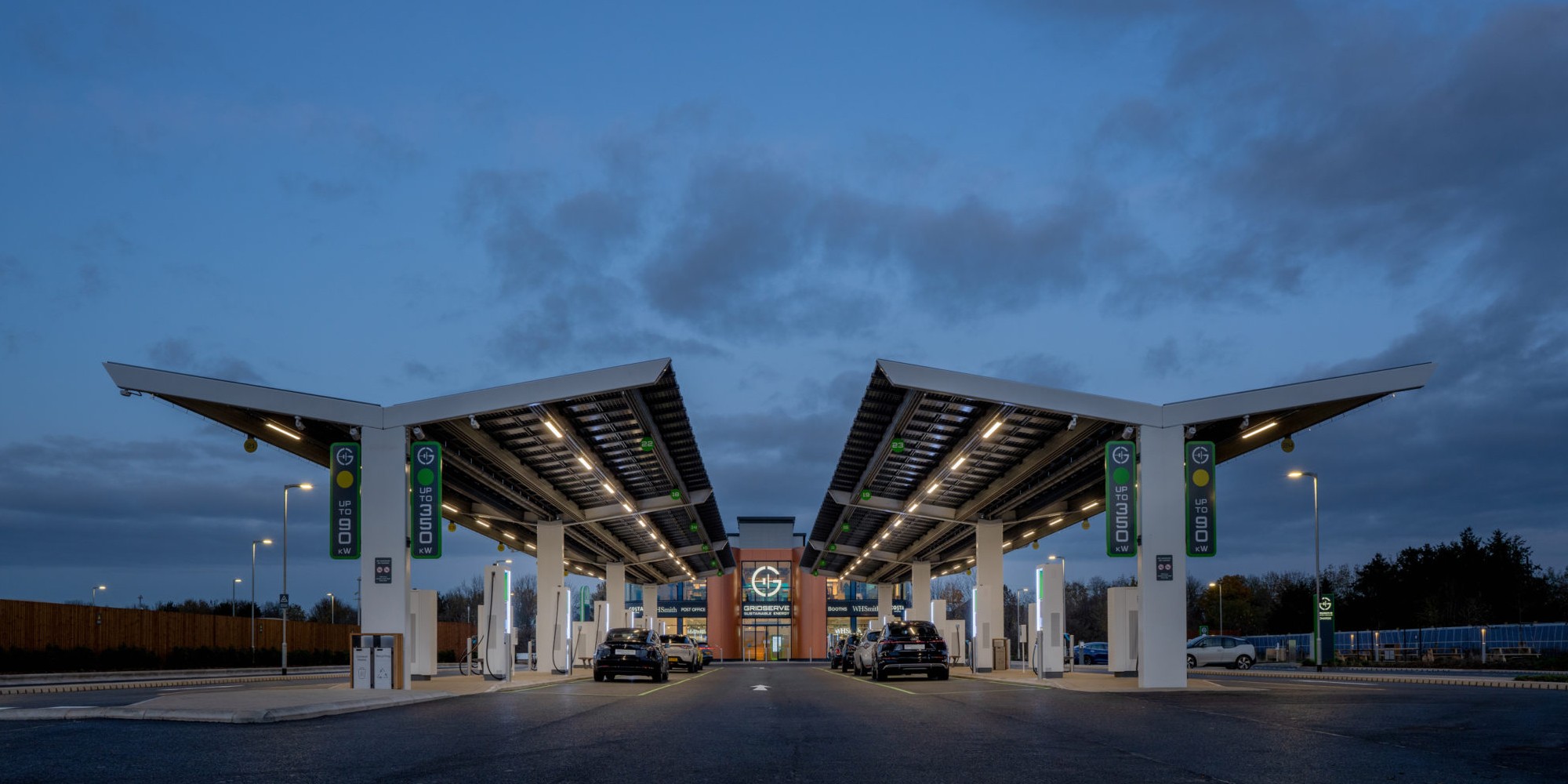The photograph captures a dusk scene at an electric car charging station, taken in a rectangular frame with a light blue sky gradually darkening under the influence of various dark grey clouds. The scene unfolds under two large canopies with a V-shaped overhang, supported by white columns adorned with LED lights and large black wires. These canopies shelter multiple charging stations, about four on each side, all bustling with parked electric cars. In the center of the photograph stands a building that appears to be a convenience market, visible through the windows with multiple store shelves inside. Green signs, albeit unreadable due to their small size, hint at the building's commercial nature. The periphery of the image reveals street lights, a wooden fence on the left, and a combination of storage containers or fences on the right. Adding to the scene's depth, trees are visible in the distance, silhouetted against the murky sky. Prominent numbers “350” and “90” alongside a 'G' on a central light fixture punctuate the functionality of this well-lit, busy electric charging station.